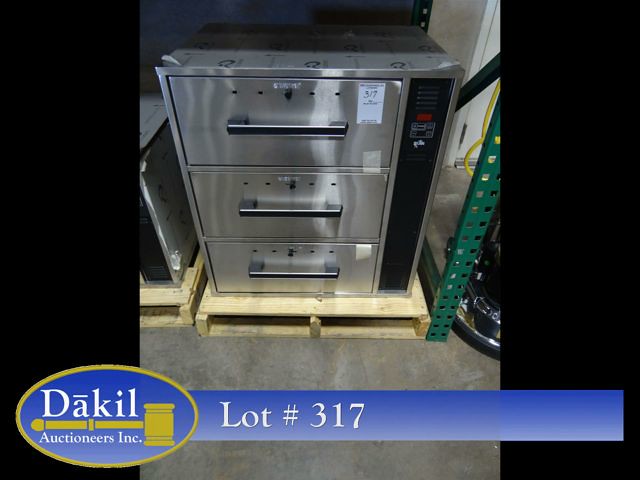The image depicts a stainless steel appliance, possibly an oven or microwave, characterized by its cube shape and three front-facing drawers, each secured with tape and featuring black handles. A white label on the top-left drawer displays the number "3-7." Adjacent to the drawers, on the right, is a vertical black bar that extends from top to bottom, possibly housing a fingerprint sensor or another functional component. At the top of this bar is a vent. The entire unit rests on a light yellow wooden pallet, positioned on a gray stone floor, and is part of a metal shelving system. Prominently displayed at the bottom of the image is a light blue line with an oval encasing the words "Dack Hill," surrounded by a gold ring. Beneath this logo is an image of a judge's hammer alongside the text "Auctioneers Incorporated," followed by "lot number 317," indicating that the item is up for auction.